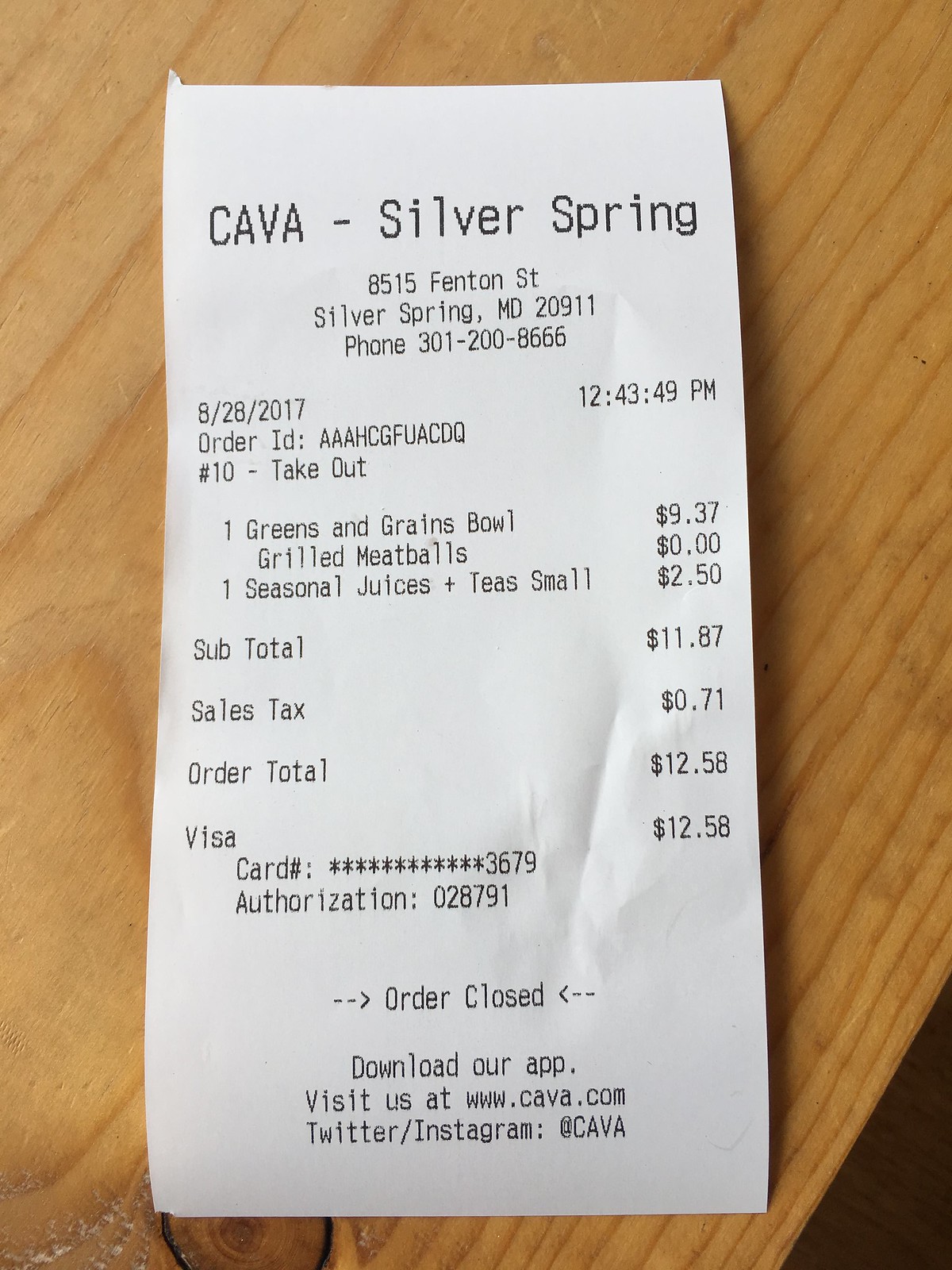This close-up photograph features a shopping receipt placed on a brown wooden surface, which appears to be either a table or a chair. The receipt, stark in its black and white color scheme, distinctly displays the title "Kava Silver Spring," indicating that the purchase was made at a restaurant named Kava located in Silver Spring. The image, devoid of any other objects or colors, directs full attention to the detailed print on the receipt. According to the document, the order was a takeout placed in August 2017, consisting of a greens and grains bowl with grilled meatballs, as well as a seasonal juice and tea. The photograph captures the simplicity and texture of the wooden background, contrasting with the clean white paper of the receipt.